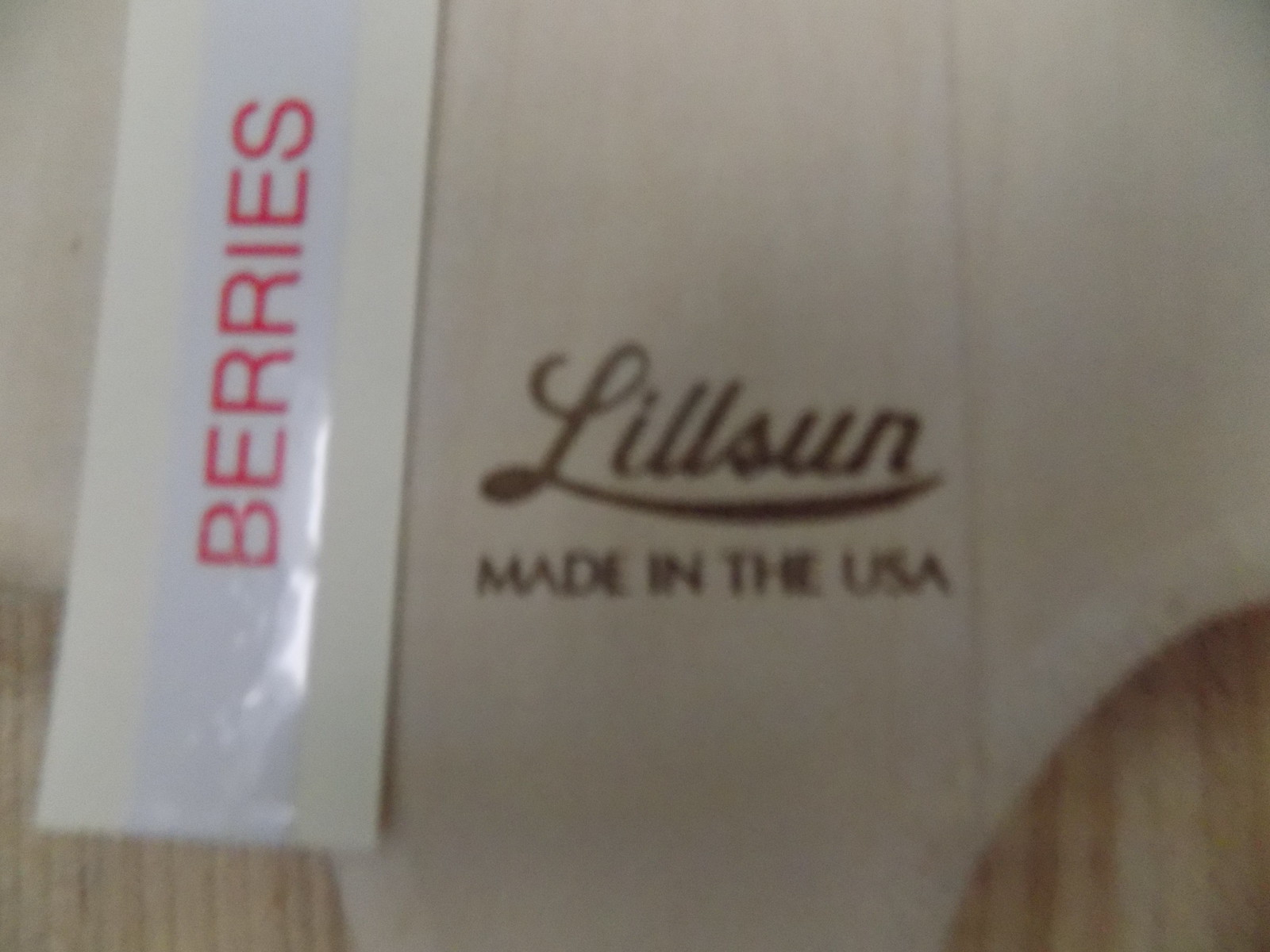This overhead photo, though slightly blurry, captures a detailed scene centered around some writing. On the left side of the image, there is a strip of white paper extending vertically from the bottom to the top with the word "BERRIES" boldly printed in red, all caps font. This white strip is backed by a light cream-colored piece of paper, adding a subtle contrast. The entire setup rests on a surface that features the word "LILSUN" written in cursive, accompanied by the phrase "Made in the USA." The precise nature of the item depicted in the photo is uncertain, though it is speculated to be a cutting board or cutting surface.